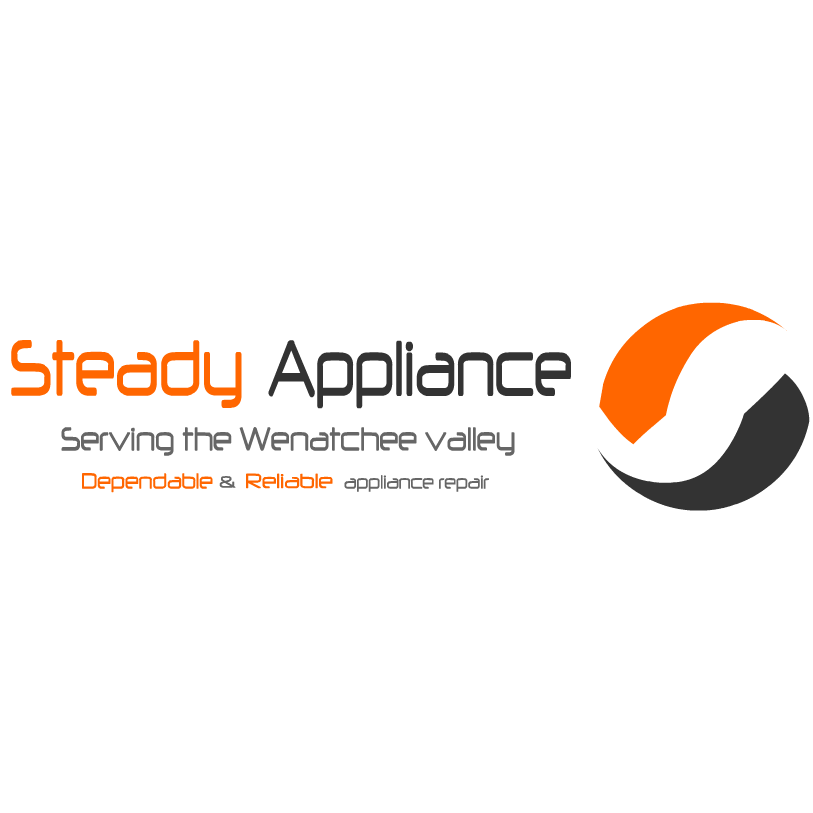This business logo, set against a plain white background, features the words "Steady Appliance" prominently. "Steady" is in striking orange letters, while "Appliance" is in bold black. Below this, in lighter gray letters, the phrase "Serving the Wenatchee Valley" is displayed. Further down, "Dependable" and "Reliable" appear in orange, with the ampersand "&" between them depicted in black. Beneath these, the words "Appliance Repair" are shown in black letters. To the right of the text, there is a symbol resembling the stripes of a volleyball, composed of two curved arrows that form a sphere-like shape: the upper arrow is orange and the lower one black, using the white background to complete the spherical appearance. The overall design is clean and professional, emphasizing the company's dependable and reliable service in appliance repair.